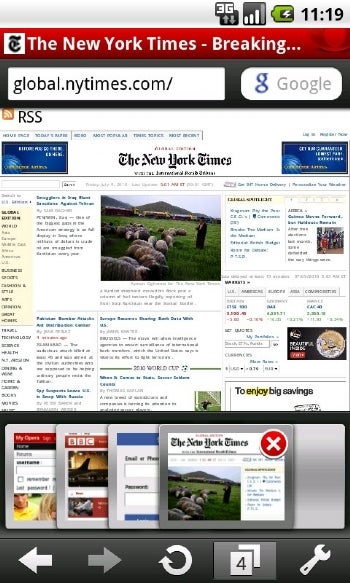Caption:  
A cell phone screenshot displaying a New York Times breaking news alert. Starting from the top right, the image shows several status icons: the 3G icon, cell phone reception bars, battery indicator, and the current time of 11:19. Just below these indicators, there is a red banner with the words "Breaking News" and the white New York Times logo on the left. The website address "global.nytimes.com" is centered in a white box, followed by the Google icon on the right. Below the web address is the RSS feed icon and label. The main content of the screenshot features the New York Times front page, displaying a prominent article accompanied by an image of a man in a black coat standing in front of a flock of sheep grazing in a green, grassy field.